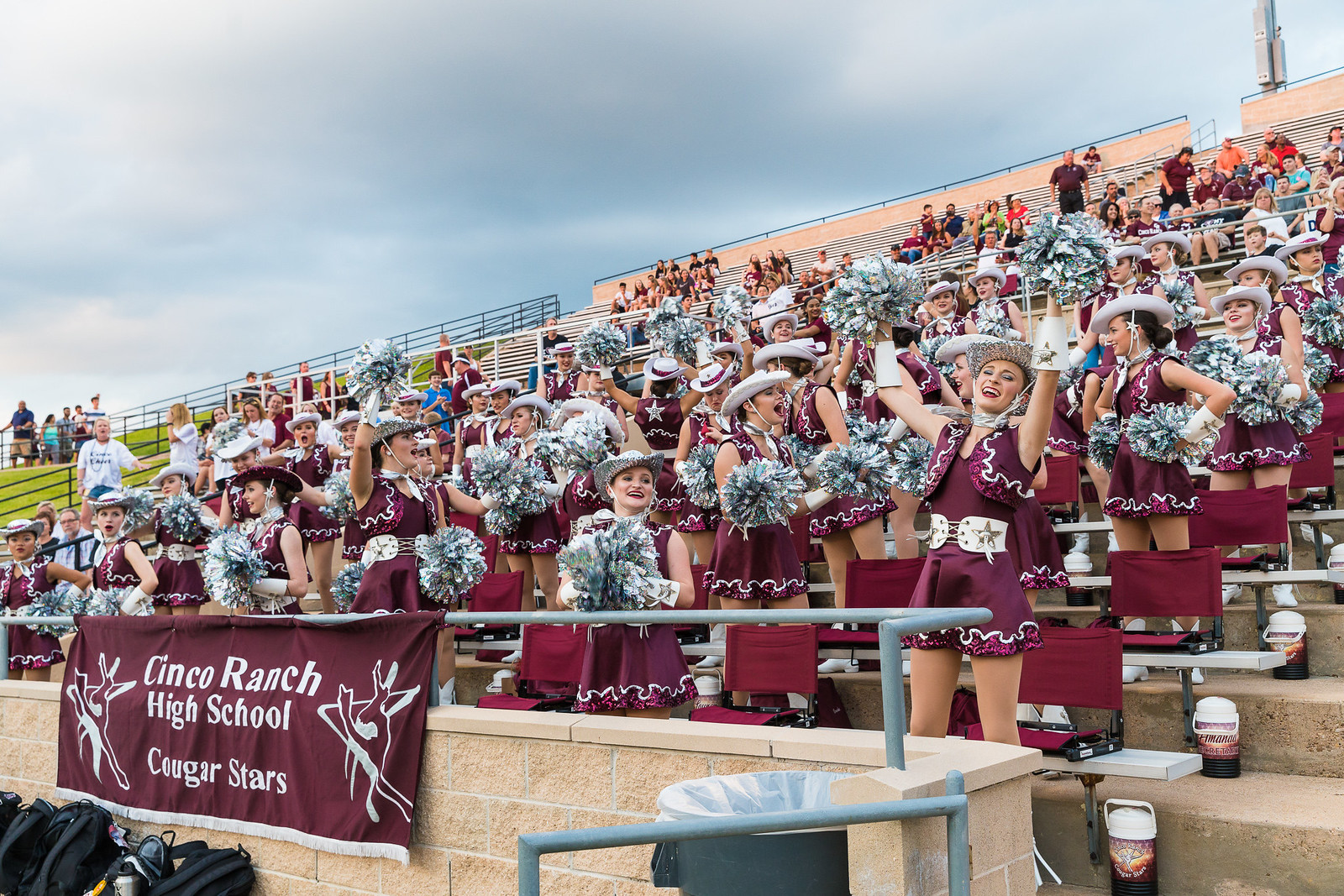The image portrays a group of women dressed in matching, dark burgundy short dresses adorned with white ruffles. They are wearing white hats tied under their chins and holding sparkly bouquets, resembling pom-poms. These women are seated in metal bleacher stands, bolted into stone steps, looking like cheerleaders in cheerleader versions of cowboy outfits. The setting appears to be a large stadium, with more people visible in the higher rows. A prominent burgundy banner in front of them reads "Cinco Ranch High School Cougar Stars." There are also bags and a trash can noticeable under the banner.